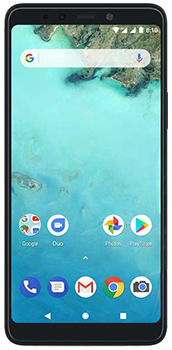This image showcases a sleek black cell phone with a black bezel encompassing the entire device. At the top section of the phone, a small speaker and microphone hole are visible. The screen displays a vivid wallpaper featuring a picturesque beach scene with crystal-clear water. In the top right corner of the wallpaper, a piece of land protrudes into view, while the middle and bottom sections prominently display the expansive ocean. Additionally, a solitary island is noticeable towards the left-center of the image.

At the top of the screen, several status icons can be seen, including indicators for Wi-Fi connectivity, signal strength, and battery level. Below these icons lies a Google search bar, marked with a "G" symbol on the left and a microphone icon on the right. 

The bottom section of the home screen contains a row of four apps: Google, Duo, Google Play, and an unidentified app. Beneath this row, there is another set of five app icons: the phone app, messaging app, Google Mail app, Google search app, and again the phone app. 

In summary, this is a black cell phone displaying a serene beach wallpaper and an organized array of application icons, providing a glimpse into the device's user interface.